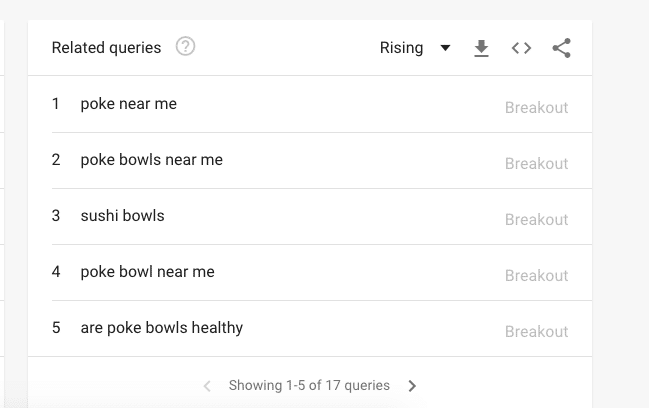### Image Caption

The image displays a search analytics dashboard with a grayish-blue background. 

- **Top Left Section**: 
   - The heading "Relative Queries" is displayed in black text.
   - A gray circle featuring a question mark icon is also present next to the heading.

- **Right-Hand Section**: 
   - The word "Rising" accompanied by a drop-down selection option is located near the top.
   - Just beneath this, there is a gray arrow pointing to a line, alongside a set of left and right navigation buttons. 
   - Also visible is an icon resembling three-fourths of a triangle with circles at each point.

- **Left-Hand Column**: 
   - The numbers 1 through 5 are listed vertically.
   - Next to each number, specific search queries are listed: 
      - 1. Poke near me 
      - 2. Poke bowls near me
      - 3. Sushi bowls
      - 4. Poke bowl near me
      - 5. Are poke bowls healthy?

- **Right-Hand Column**:
   - The word "Breakout" appears in gray text next to each query, indicating significant increases in search popularity.

The overall layout and design of the dashboard offer a comprehensive view of trending search queries related to poke bowls.